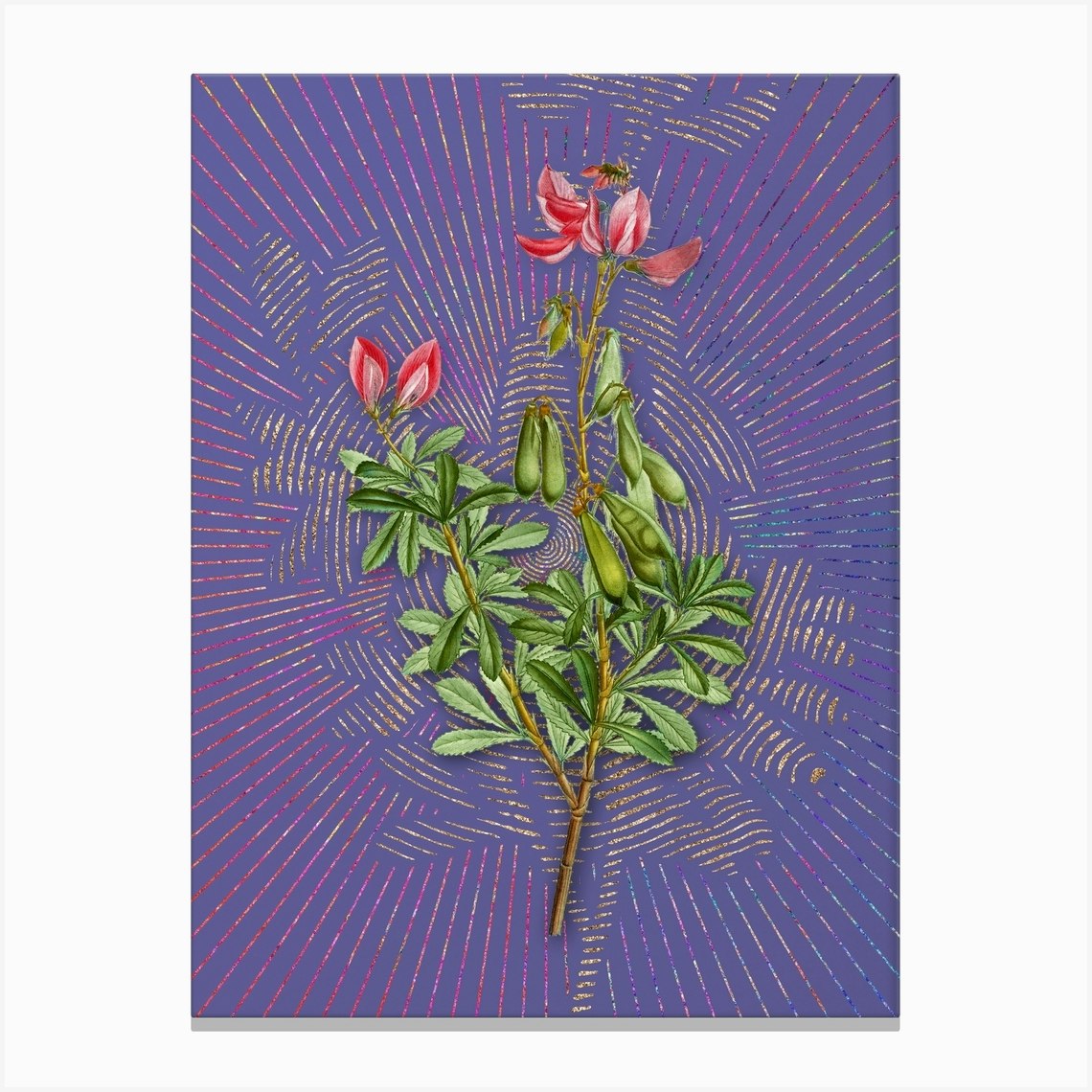This is a detailed photograph of a flowering plant set against a purple background adorned with light red lines that create an intricate pattern. The focal point is a plant with two woody stems radiating from a central base. The left stem extends at an angle, while the right one stands taller. The plant is adorned with a multitude of medium green leaves, approximately 20 to 40 in number. The stems host a combination of pinkish-red flowers and buds, with four fully opened blossoms and several more buds poised to bloom. Some of these buds appear like green pea pods, with one pod revealing rounded, bean-like seeds. Notably, at the top of the taller stem, a honeybee can be seen attempting to access the pollen at the flower's center. The harmonious interplay of the plant's natural beauty and the artistic, patterned background creates a captivating visual.